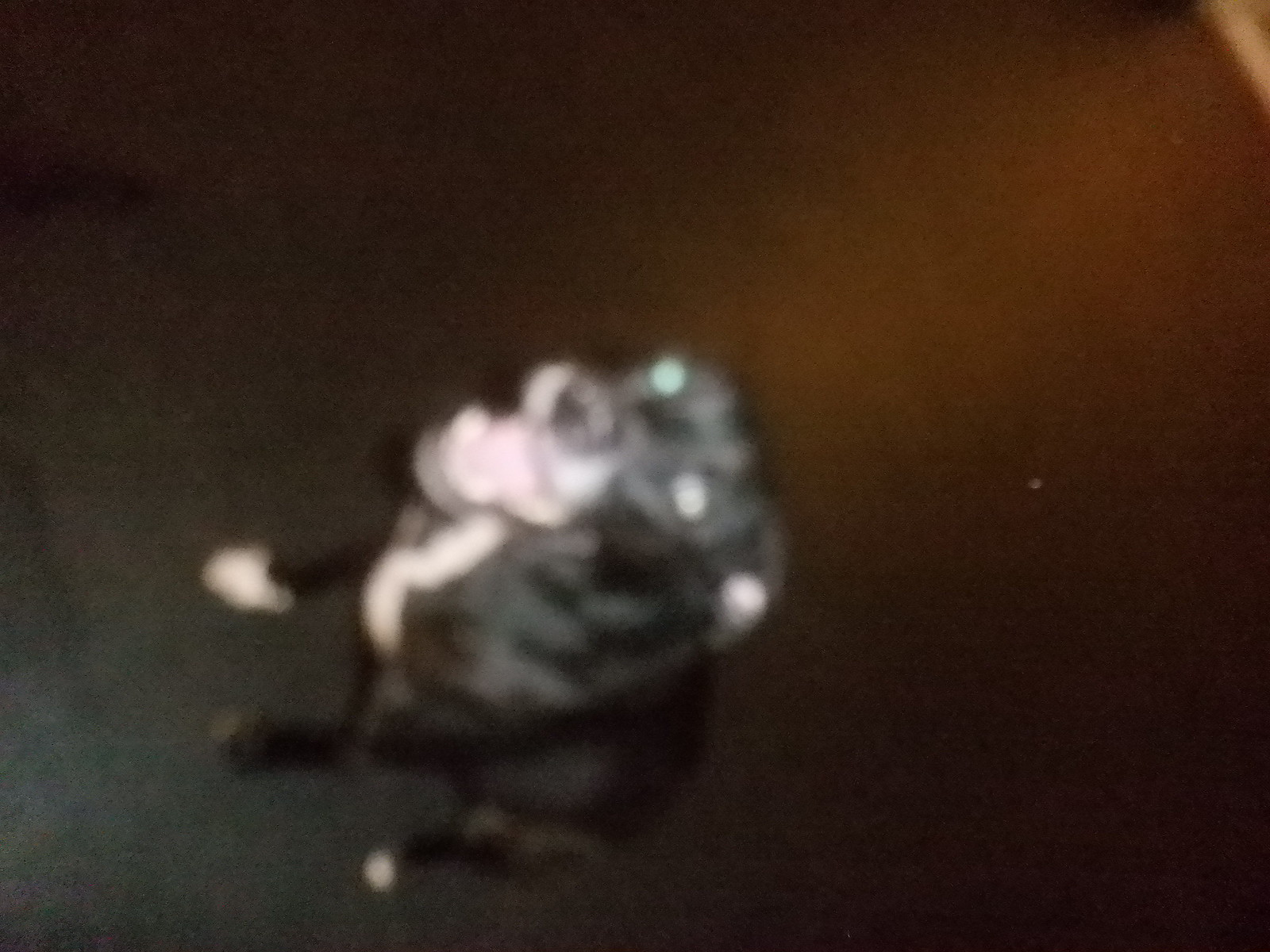This image is a blurry, close-up photograph of a black and white dog, oriented sideways, making it look as if the dog is standing on the left-hand side of the photo. The dog appears to be sitting and looking up at the photographer, with its mouth open in what resembles a dog smile, revealing part of its bottom teeth. The dog's right eye catches the light, giving it a greenish glow.

The dog's fur is predominantly black with distinctive white markings: a white-tipped right front paw, a white-tipped left hind paw, a patch of white on its snout and chest, and a touch of white on the inside of its left ear. There is also a noticeable white stripe running from its neck down its chest.

The background of the image is hard to discern due to the blur. The right half (or top of the original orientation) is a red-brown color, possibly indicative of a wall or carpet, while the bottom corner (or left corner in the original orientation) is black, suggesting an area of dark flooring or shadow. There is no text in the image, and the overall photograph gives a sense of an oddly angled, momentary snapshot.